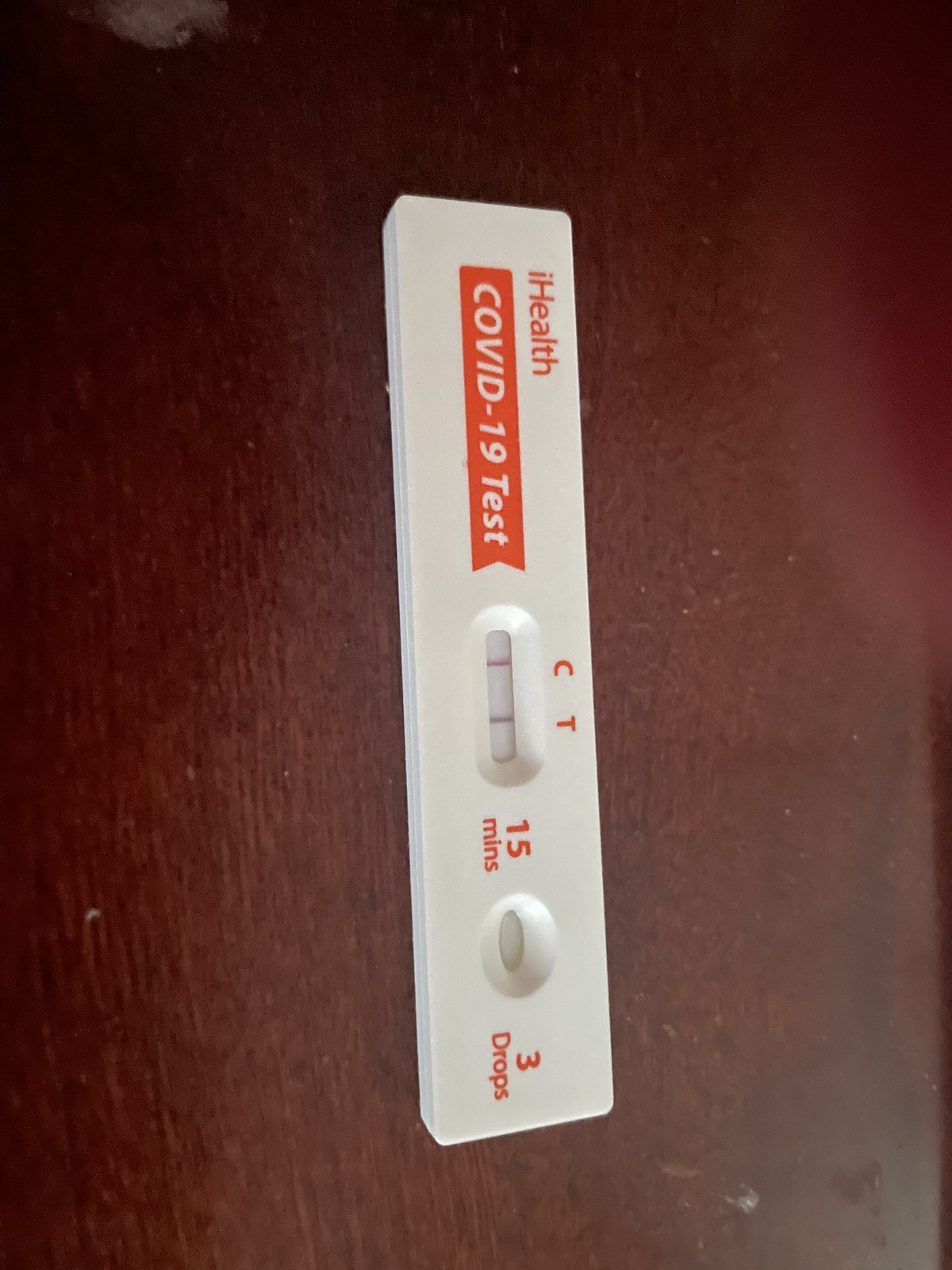A close-up image captures an iHealth COVID-19 test lying on a dark brown, slightly dirty table with some smudges in the bottom right corner. The photo is taken with a flash, which prominently highlights the test against the brown background. The COVID-19 test kit is positioned horizontally, turned 90 degrees to the right, requiring viewers to tilt their heads to read it properly. The white test strip features red-orange lettering that reads "COVID-19 Test." The test section includes the letters "C" and "T" with two lines indicating a positive result as there is a line under the "T." Additional text indicating "15 minutes" is positioned to the right, alongside an area marked for entering three drops of a solution.